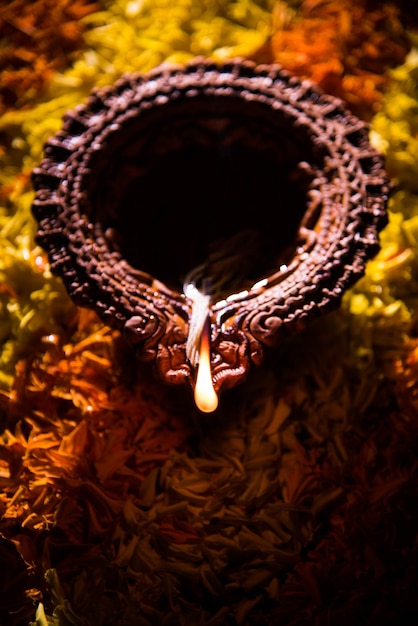The image depicts a computer-generated photograph of a circular, dark brownish-red object prominently featured in the center. The object has intricate, rope-like textures and appears to resemble a bowl with detailed, woven edges. One part of the object is pointed like a spout, from which an off-white liquid is seen dripping downward. The background is blurred, featuring dark yellow to orange-red organic textures that look like leaves or flower-like substances. The lighting in the background creates deep shadows, especially in the lower and right corners, adding to the depth of the scene.